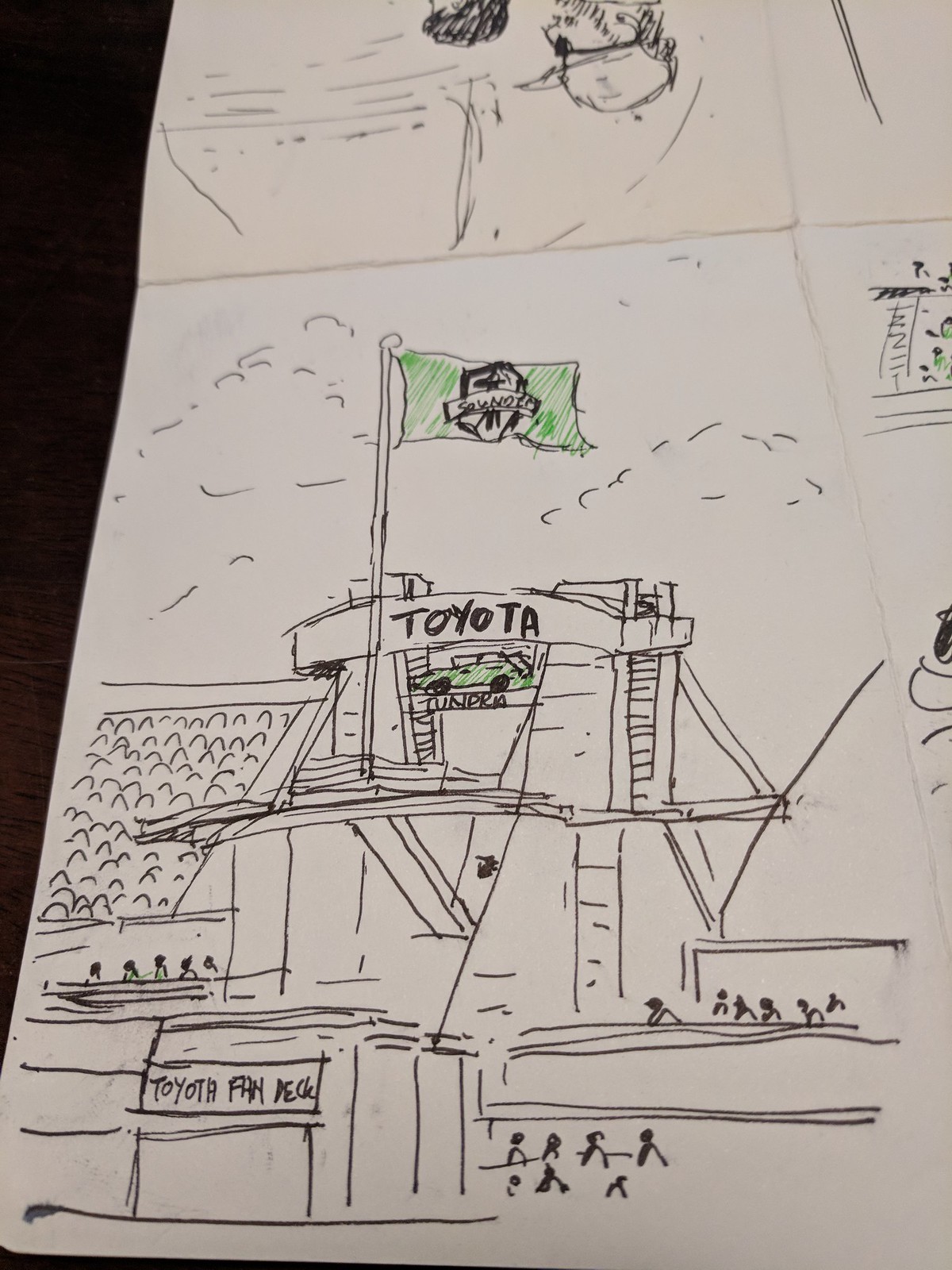The photograph showcases several sketches laid out on a table, with the focal point being a detailed drawing of a three-tiered structure possibly located in a stadium. This main sketch is primarily done in black ink and is accented with green colored pencil for additional details. It features a large flagpole on the top tier, flying a green pennant with a black logo. Surrounding the flagpole is a gently arched roof supported by structures resembling bridge towers. There's a platform with the word "Toyota" visible alongside what looks like the name of a vehicle model, possibly "Tundra," though it's obscured. A sports car, also colored in green, is depicted beneath this text. 

The lower tiers of the structure show rows of small, half-line sketches that appear to represent spectators. At the base, there is a large entryway labeled "Toyota Fan," indicating the main entry to the stadium-like structure. Adjacent to the central drawing, the edges of other sketches are visible: one showing the top of a person's head wearing a ball cap and sunglasses, another sketch displaying minimalistic ink lines, and a third partially colored with green and black ink. The background surface appears dark, providing contrast to the sketches.